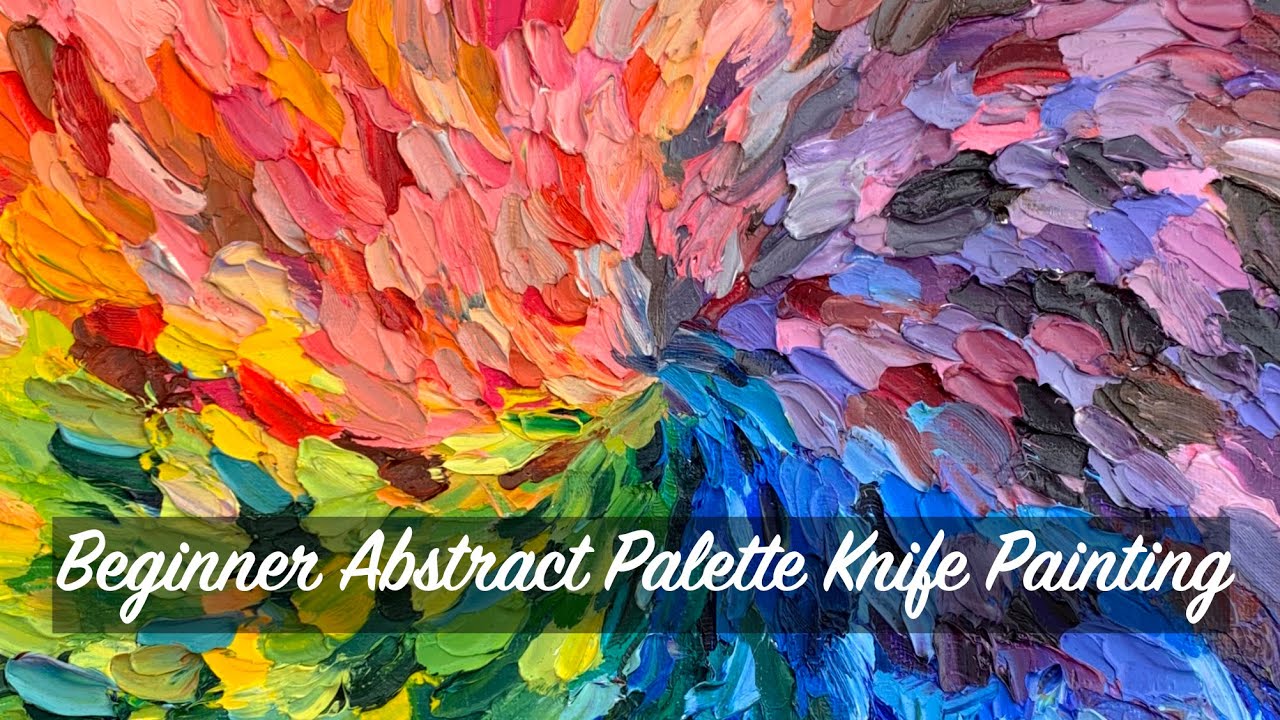The image is a captivating example of a beginner abstract palette knife painting, showcasing a vibrant array of colors and textures. The painting features a dynamic, swirling composition, starting from the center and radiating outward in a circular pattern. The colors transition smoothly through the spectrum: red at the top, progressing to yellow, green, blue, and finally a purple-violet blend, with each hue subtly mingling with adjacent shades, creating a seamless gradient.

In the top left corner, feather-like elements in red, pink, and yellow converge towards the edge, forming a striking and cohesive section. The top right corner displays a quilt-like arrangement of tapering shapes in black, purple, blue, and pink, all converging towards the center. The bottom left corner highlights leaf-like shapes in various shades of green, swirling towards the center, adding depth and movement. The bottom right corner features blue, tapered forms meeting in the middle, enhancing the overall sense of flow and unity.

A black bar runs horizontally near the bottom of the image, containing the phrase "Beginner Abstract Palette Knife Painting" in cursive font, indicating it might be an ad for an art class or blog. This text, combined with the rich visual elements, creates an inviting and educational piece, perfect for those interested in exploring the art of palette knife painting.